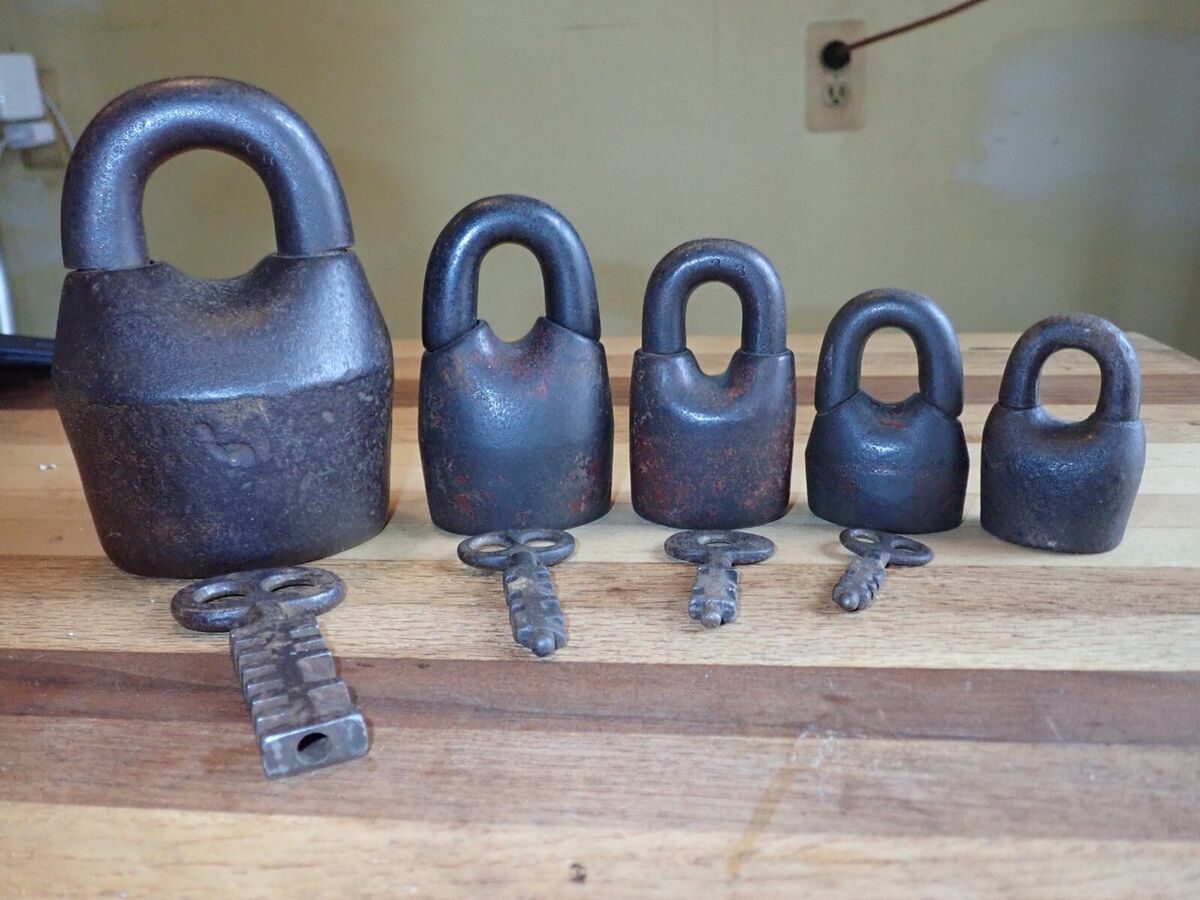The photograph depicts five vintage, iron padlocks arranged from largest to smallest on a slightly brown butcher block wood table. Each padlock, characterized by its worn, rust-speckled exterior and intricate design, exudes an air of antiquity, perhaps dating back to the early 1900s or even the 1800s. In front of the four largest padlocks, corresponding keys, some with multiple prongs, are neatly aligned, while the smallest padlock on the far right is missing its key. The backdrop of the scene includes a cream-colored wall with an outlet from which a black cord ascends. The dim lighting and visible wall outlets suggest the photo was taken inside a house.